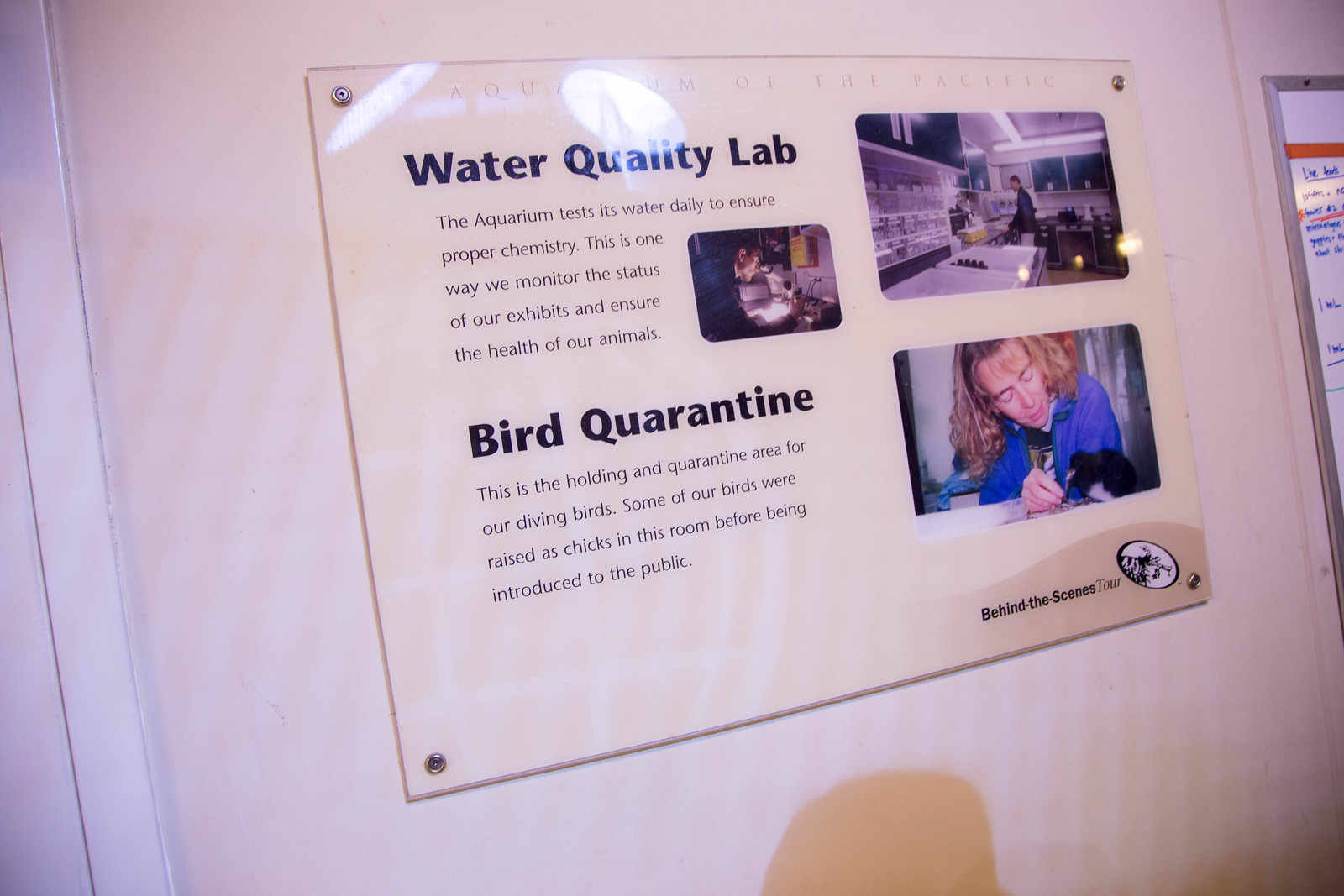The image is a glossy, rectangular plaque bolted to a white wall, titled "Aquarium of the Pacific" at the top. This informative plaque is part of a behind-the-scenes tour. It features two main sections with black text headers: "Water Quality Lab" and "Bird Quarantine."

Under the "Water Quality Lab" header, the text explains that the aquarium conducts daily water tests to ensure proper chemistry, which helps monitor exhibit conditions and ensure the health of the animals. To the right of this section, there is a photograph depicting a lab facility where a man is working, illustrating the lab activities.

Under the "Bird Quarantine" header, the text describes the holding and quarantine area for diving birds, noting that some birds were raised as chicks in this room before being introduced to the public. Adjacent to this section, there is an image showing a woman in a blue lab coat feeding a mostly black bird with a yellow beak on a table.

The bottom right corner of the plaque features a small logo that reads "Behind the Scenes Tour." The light reflection on the glossy surface partially obscures some details, but the key information remains clear.